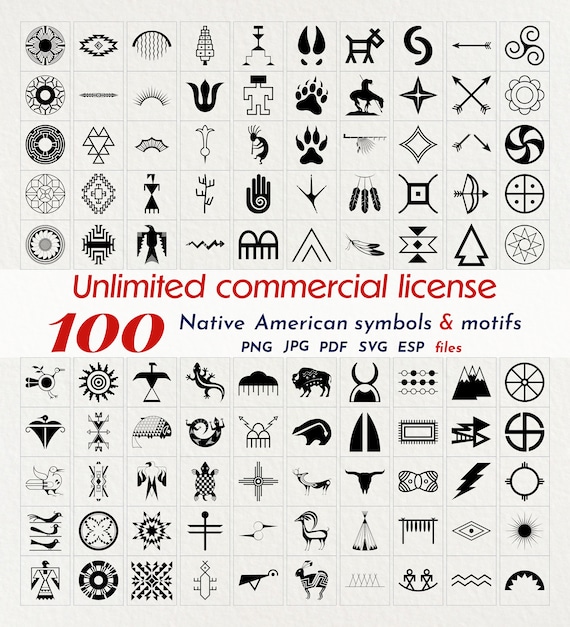The image displays an assortment of 80 different black and white Native American symbols and motifs, arranged in a grid of 10 columns and 8 rows. Each symbol is displayed within a small square against a white background. The text in the center of the image prominently states "Unlimited Commercial License 100 Native American Symbols and Motifs" in red and blue letters. It further mentions that the symbols can be saved in various file formats such as PNG, JPG, PDF, SVG, and ESP. The symbols encompass a variety of Native American cultural elements including circular designs, plants, arrows, lightning bolts, animals like buffalo, rain clouds, suns, and various religious symbols. The only color present in the image is within the text, using red for "Unlimited Commercial License 100" and "Files," and blue for "Native American Symbols and Motifs" and the file extensions.